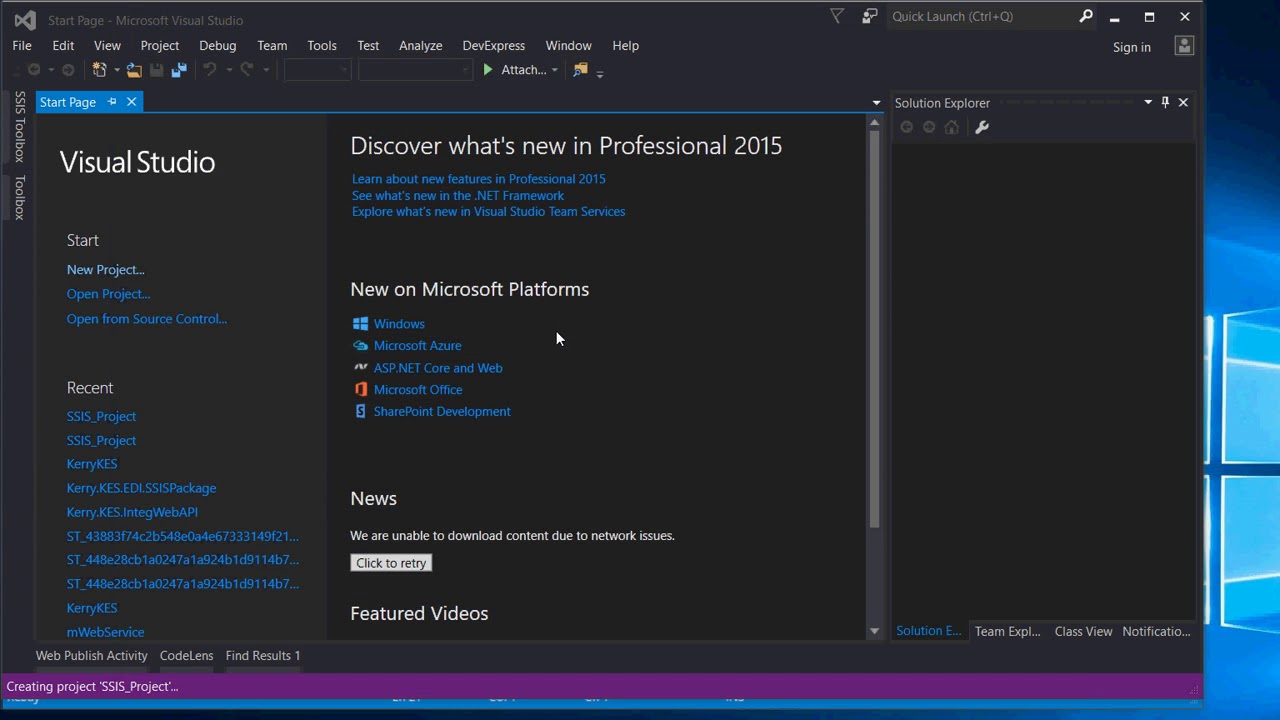A user has opened Microsoft Visual Studio 2015 on their Windows desktop, visible due to the partially displayed generic Windows logo background. The Visual Studio window is not maximized and reveals several standard interface elements. The application is set to dark mode, featuring a black background with contrasting blue font. 

The start page tab is open, presenting options including "New Project," "Open Project," "Open from Source Control," and a list of recent projects, indicating this is not the user's first time using the software. The central pane highlights a section titled "Discover What's New in Professional 2015," showcasing products such as SharePoint and Azure. To the right, the Solution Explorer pane is empty, indicating no project is currently loaded.